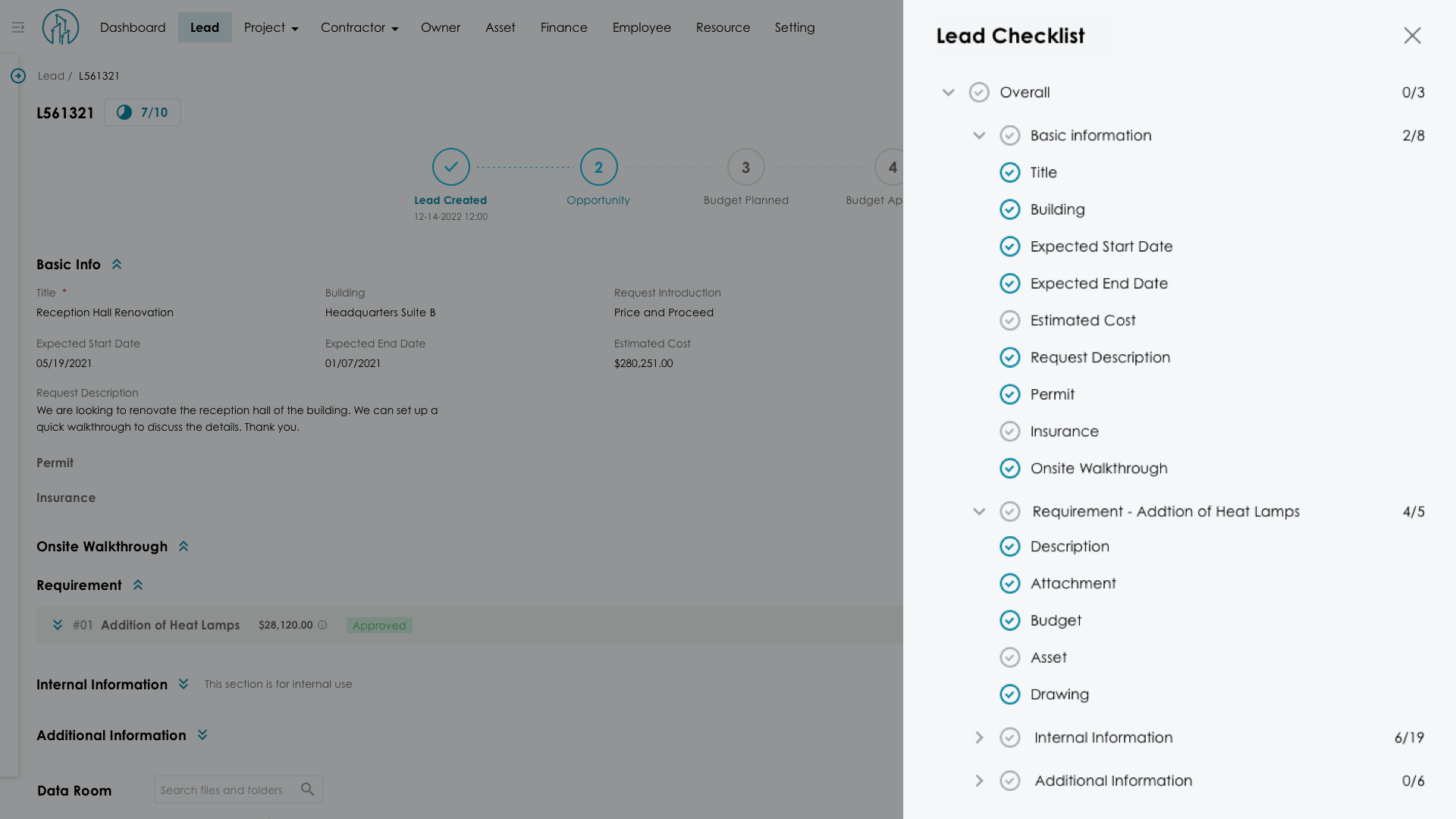This is a detailed screenshot of a lead checklist interface. On the upper left-hand side, there's a distinctive logo featuring triangular-style gems within a blue or teal circle. The navigation bar at the top includes options such as Dashboard, Lead, Project, Contractor, Owner, Asset, Finance, Employee, Resource, and Setting, with the 'Lead' page currently highlighted in a blue box.

The lead in focus is identified as Lead L561321, repeated twice for clarity. Below the lead identifier, there is a graph indicating progress with a score of 7 out of 10, and a section labeled "Leads Created," though the exact number isn't legible.

The main content area is divided into several sections. It includes:
- Basic Info
- On-Site Walkthrough
- Requirement
- Internal Information
- Additional Information
- Data Room

On the right-hand side of the screen, a detailed lead checklist is displayed with an 'X' in the top right corner for closing the menu. A drop-down menu labeled 'Overall' precedes the checklist content.

The checklist is organized as follows:
- Basic Information: 2 out of 8 completed
  - Title: Checked
  - Building: Checked
  - Expected Start Date: Checked
  - Expected End Date: Checked
  - Estimated Cost
  - Request Description: Checked
  - Permit: Checked
  - Insurance

- On-Site Walkthrough: Checked

- Requirement: 4 out of 5 completed
  - Description: Checked
  - Attachment: Checked
  - Budget: Checked
  - Asset: Checked
  - Drawing

- Internal Information: 6 out of 19 completed

- Additional Information: 0 out of 6 completed

Overall, the screenshot provides a comprehensive view of the lead's progress and necessary information stages, highlighting both completed and pending items systematically.